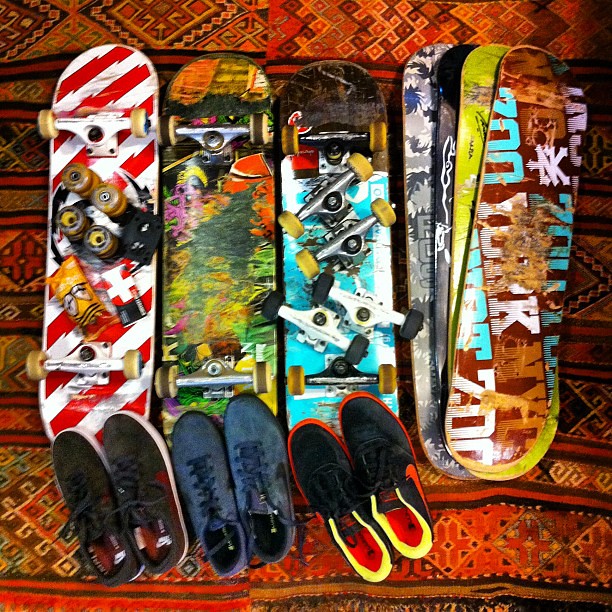The image is a detailed photograph showcasing an array of skateboards and shoes arranged on a vibrant, geometric-patterned rug with shades of black, orange, gold, yellow, and green. From left to right, the scene begins with a skateboard featuring a red and white candy cane stripe pattern, accompanied by a set of wheels and a plastic package on top, and a pair of black tennis shoes positioned at the bottom. Next to it, another skateboard displays a dynamic splattered paint pattern with a hint of a green tree in the middle, below which rests a pair of black shoes. The third skateboard exhibits a blue and white background with a set of disassembled wheels and metal attachments, matched by a pair of black tennis shoes with red insides and yellow borders. On the far right, there is a somewhat chaotic pile of four skateboard decks without wheels, spread slightly apart, each with distinct graphic patterns including shades of tan, blue, white, lime green, black, navy, gray, silver, purple, red, yellow, and orange. The entire ensemble, including the footwear and skateboards, is meticulously placed on top of the eye-catching rug, creating a detailed and visually engaging composition.